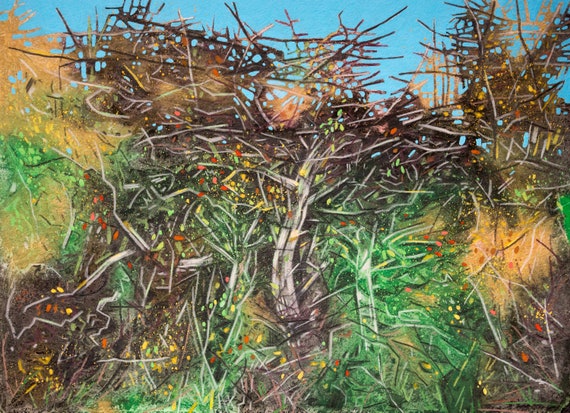This image captures an outdoor scene depicting a chaotic tangle of twisted, broken branches and dead gray sticks, resembling a hay bale. The branches are predominantly brown and appear lifeless. Among the disarray of dead wood, vibrant splashes of color punctuate the scene. Yellow and green splashes, possibly stylized leaves, intermingle with occasional red splotches that might represent berries. In the background, patches of blue sky peek through, juxtaposing the scene's overall mixture of decay and brief bursts of color. It presents a stark and evocative contrast, blending elements of nature's decline with vivid hints of life.